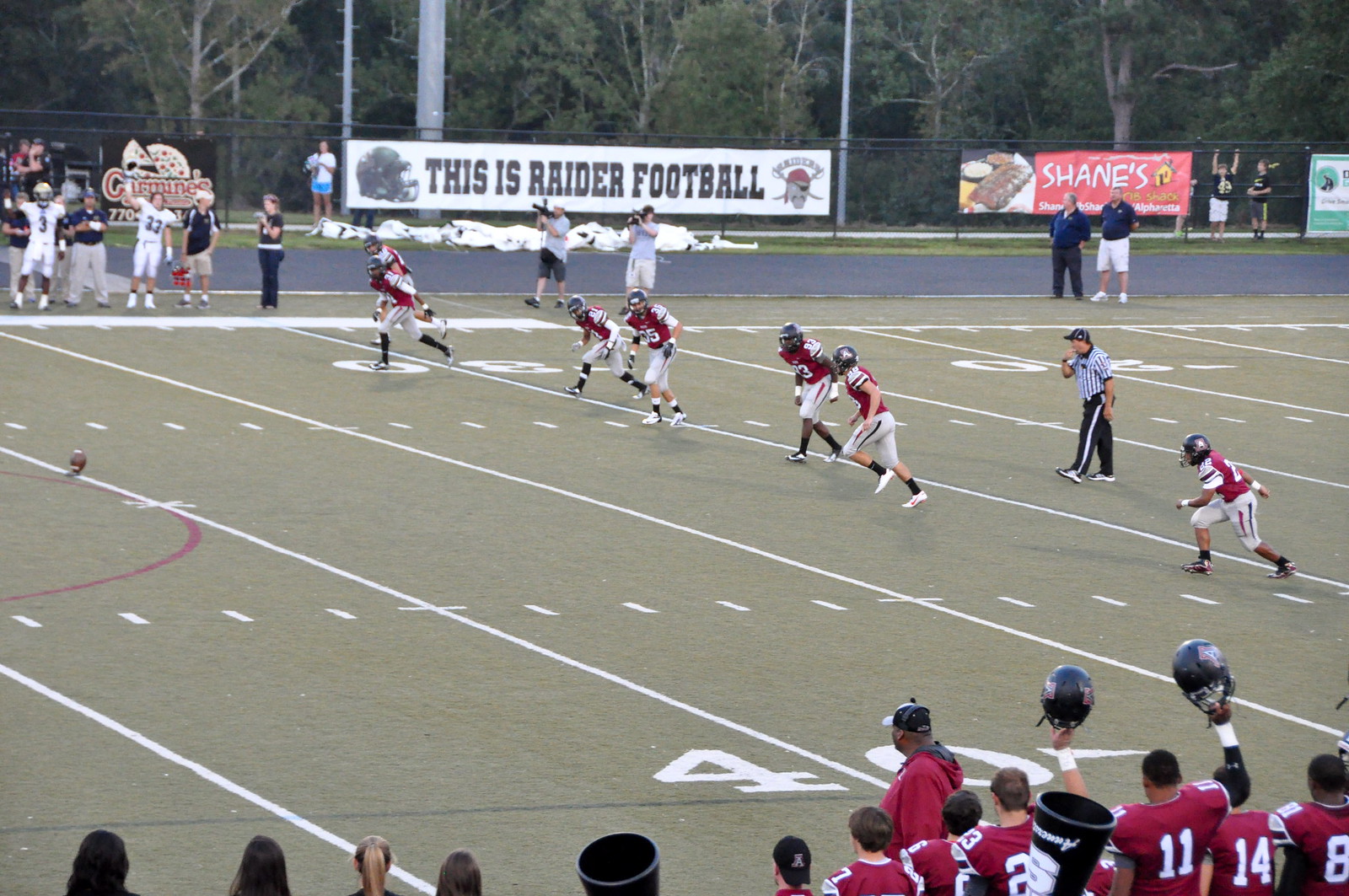This horizontally oriented outdoor photograph captures an exhilarating moment of an American high school football game. Centered on the gridded, dull green field marked with white lines, the image features a team in red jerseys, gray pants, and black helmets positioned around the 30-yard line, poised to kick off. A line of players is gearing up to sprint downfield, encapsulating the anticipation of the kickoff. On the right side, a referee is captured mid-stride, seemingly ready to blow his whistle.

In the foreground, along the near edge of the field, members of the same team also in red, some raising their black helmets, can be seen cheering on their teammates. The background layers the excitement with additional visual details: a sleek black chain-link fence lined with banners. One prominent banner reads, "This is Raider Football," accompanied by a football helmet and a pirate symbol. Another banner, promoting Shane's Restaurant, features an appetizing image of ribs or steak.

Beyond the players and banners, the scene is softened by lush green trees and more spectators scattered along the sidelines, all contributing to the vibrant, communal atmosphere of high school football.